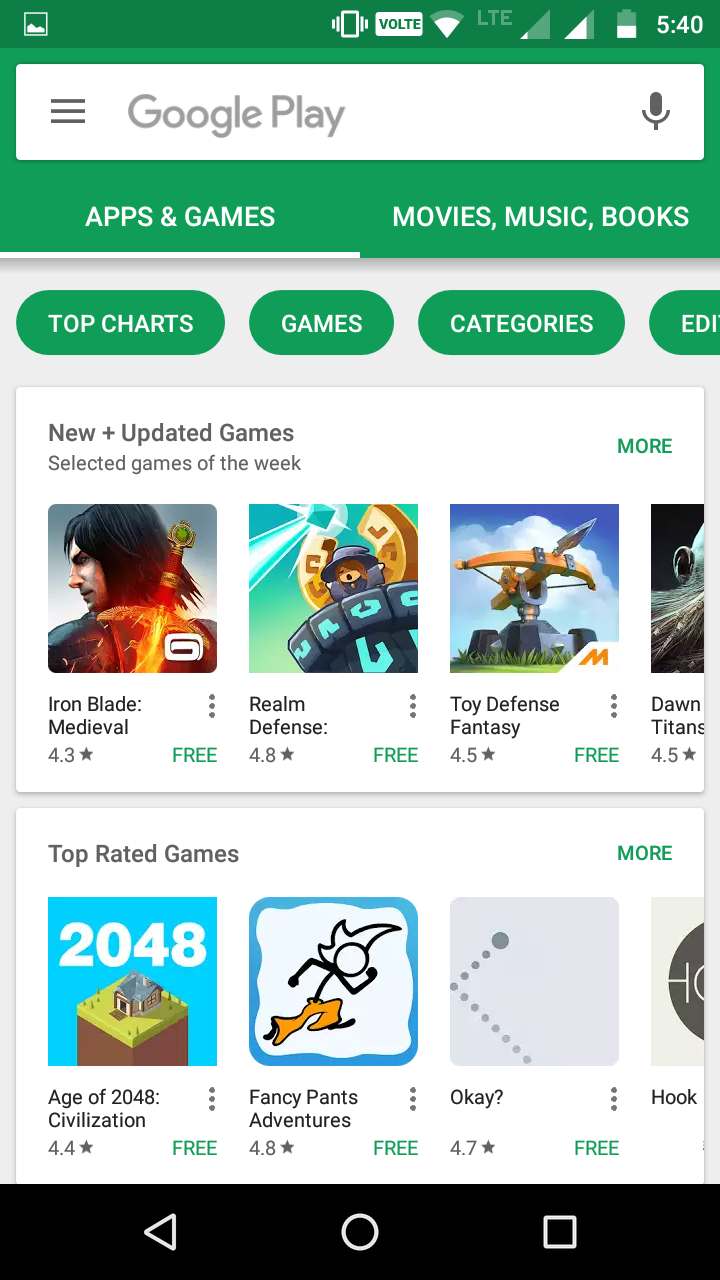Screenshot of a Google Play Store Page

The screen capture showcases a page from the Google Play Store, prominently featuring green branding at the top with the "Google Play" logo. Below the logo, navigation tabs for "Apps," "Games," "Movies," "Music," and "Books" are displayed, allowing users to toggle between various content categories. The user's status bar is also visible, indicating the time, signal strength, and remaining battery charge.

The primary focus of the screenshot is on the "Top Charts" and "New and Updated Games" sections, listing several mobile games available for download. 

Highlighted games include:
- **Iron Blade: Medieval Legends**: Rated 4.3 stars, this game is free to download.
- **Realm Defense**: A child-friendly game rated 4.8 stars, also free.
- **Toy Defense Fantasy**: Another free game displayed in this section.
- **Going Titans**: Not explicitly detailed but present in the list of free games.

Further down, the "Top-Rated Games" section showcases:
- **Age of Civilizations**: Rated 4.4 stars and free to download.
- **Fancy Pants Adventures**: Rated 4.8 stars and also free.
- **Hook**: Part of the displayed top-rated games.

Overall, the screenshot provides a detailed view of various game options available on the Google Play Store, emphasizing free games with high user ratings.